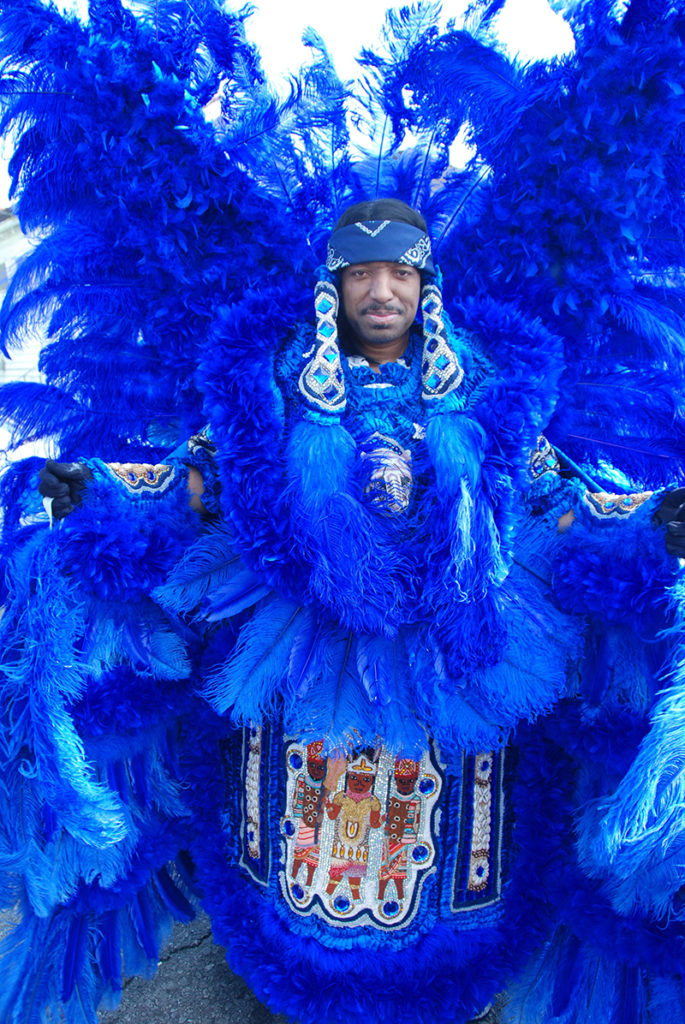The image features a black man dressed in an elaborate, festive costume predominantly adorned with blue feathers and ornate decorations. His attire includes a large, furry cloak that extends into a dress-like garment, embellished with detailed stitching of three darker-complexioned cartoonish figures, possibly pharaohs, standing side-by-side at the bottom. These figures also wear headdresses and cloaks hinting at a possible cultural or ceremonial significance. He wears a striking headdress from which blue and white twisted braids hang, along with additional feather accents. Blue feathers not only crown his head but also extend horizontally from his sides and vertically below his waist. His arms are draped with long feathers, contributing to a grandiose, bird-like appearance. The entire ensemble suggests that he might be preparing for a traditional dance, performance, or religious festival, deeply immersed in the ritualistic ambiance conveyed by his attire.